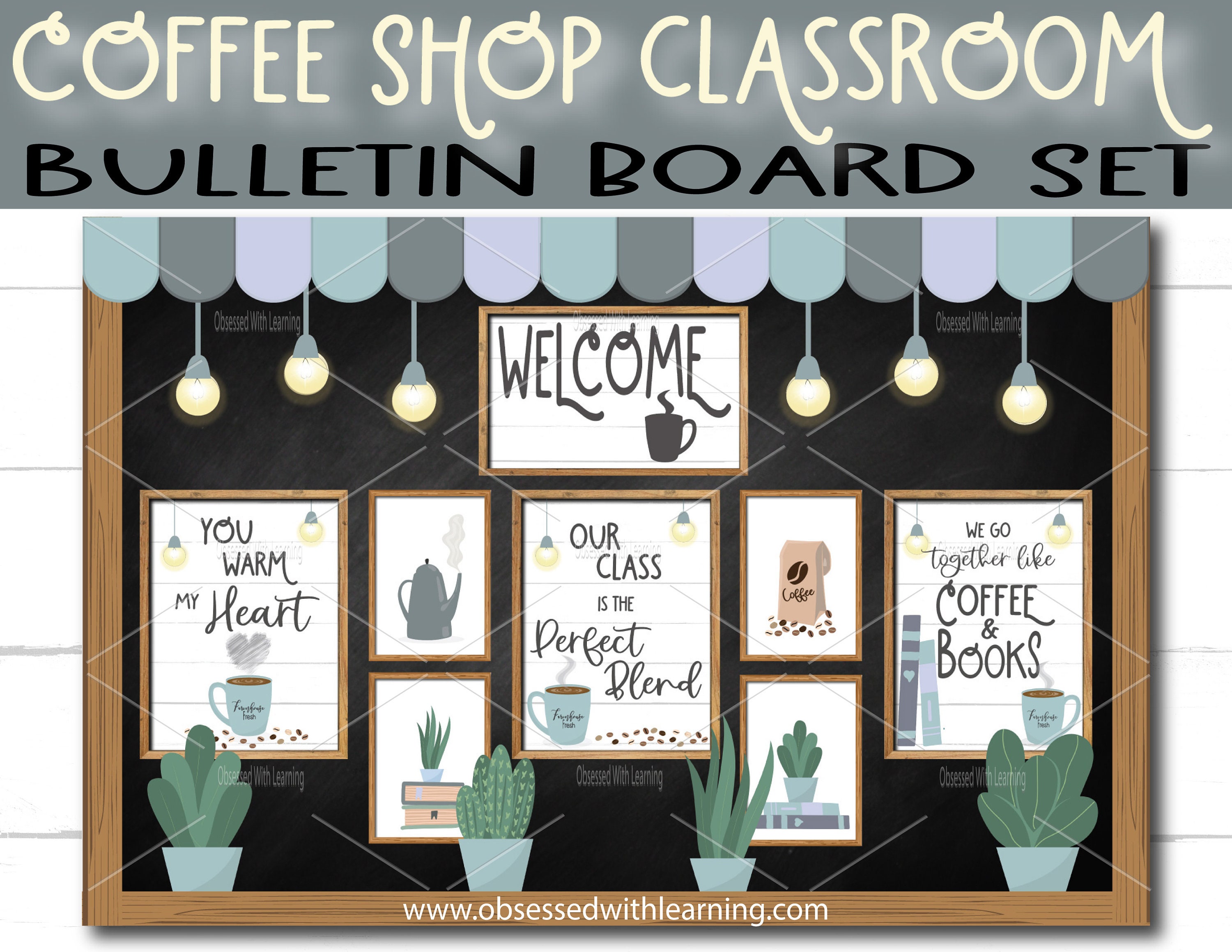This digitally created image features a detailed depiction of a Coffee Shop Classroom Bulletin Board Set, designed as a vibrant and welcoming space. At the top, a large gray banner reads "Coffee Shop Classroom" in cream letters, with "Bulletin Board Set" written in bold, black letters below it. The banner is adorned with alternating colors of light gray, dark gray, and very light purple, creating a scalloped edge, and faux lights are artfully hung from it, adding a charming touch.

Central to the image is a welcoming sign featuring a silhouette of a steaming cup of coffee, flanked by three lamps on either side. The theme of coffee is prevalent throughout, with various inspirational phrases such as "Our class is the perfect blend" paired with an image of a steaming cup of coffee on a table with coffee beans, and "We go together like coffee and books," illustrated with books and a steaming cup of coffee on a table. Another highlighted phrase is "You warm my heart," accompanied by heart-shaped steam rising over a cup of coffee.

The image also includes multiple illustrations of succulent plants, providing a fresh, green contrast to the coffee theme. Additionally, the wording "www.obsessedwithlearning.com" is featured at the bottom, tying the design together into a cohesive and inviting classroom decor piece.